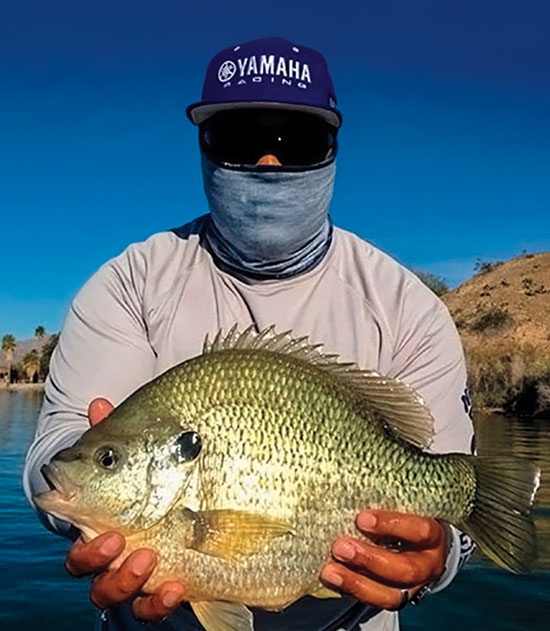In the photograph, a muscular man stands prominently in the center, holding a small, shiny greenish fish up toward the camera. The fish is wide but not thick, with slightly spiky fins along its back, small wispy side fins, and a glossy gunmetal-colored tail. The man's tan hands, sporting a wedding ring and short nails, can be seen gripping the fish firmly. He is dressed in a beige long-sleeve t-shirt, a light blue ski mask covering most of his face, and dark reflective goggles. His lips and the tip of his nose are just visible beneath the mask. He wears a Yamaha Racing blue baseball cap, distinguished by its white stitched emblem and lettering. Behind him, the sky is clear and vivid blue, with no clouds in sight. On the left, a small, arid hill extends into the backdrop, and on the right, distant palm trees dot the landscape. A calm body of water occupies the lower portion of the image, completing the tropical scenery.